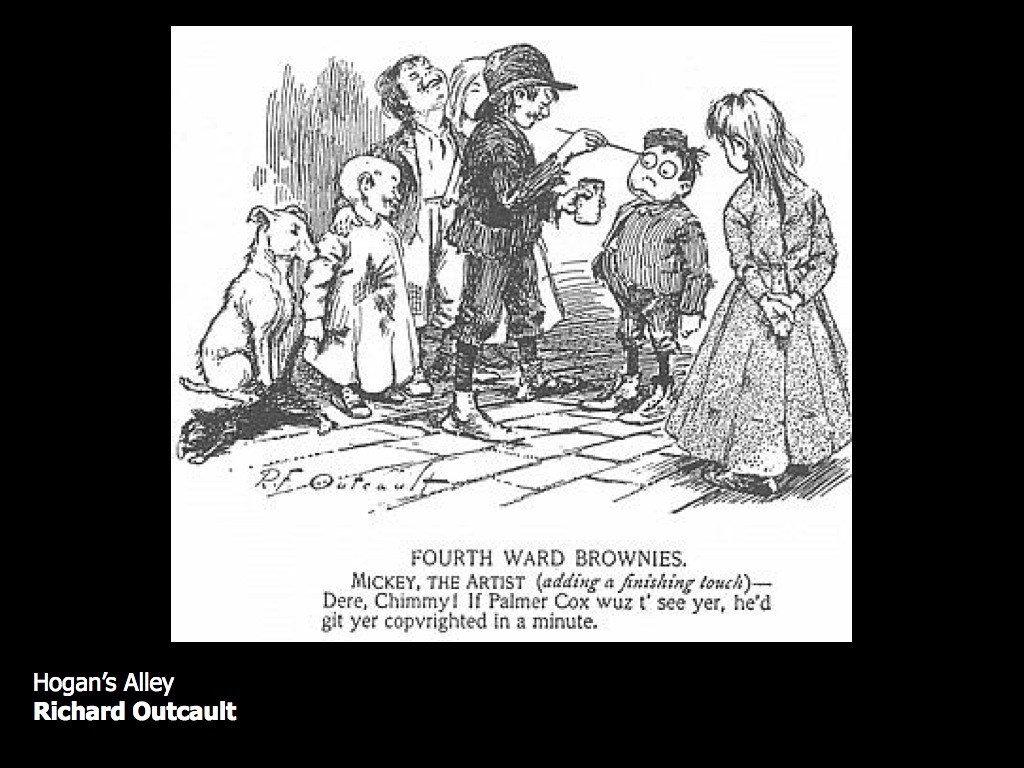The black and white cartoon illustration, framed with a plain black border, depicts a group of children standing in a cobbled field area. Central to the image is a boy with dark hair, eyes bugged out, who holds a paintbrush and a paint can, finishing drawing a face on another boy, who also has big eyes and dark hair. A girl with blonde hair, wearing a long dress and with her hands behind her back, watches intently. On the left side of the image stands a dog with light-colored fur, upright on its hind legs, near another group comprising two girls and a boy, the latter with a patch on his knee. In the background, a tree subtly frames the scene. At the bottom, text reads, "Fourth Ward Brownies, Mickey the artist, adding a finishing touch. Dear Chimmy, if Palmer Cox was to see you, he’d get you copyrighted in a minute." Adjacent to the border, at the lower left corner, "Hogan's Alley, Richard Outcault" is inscribed in white.